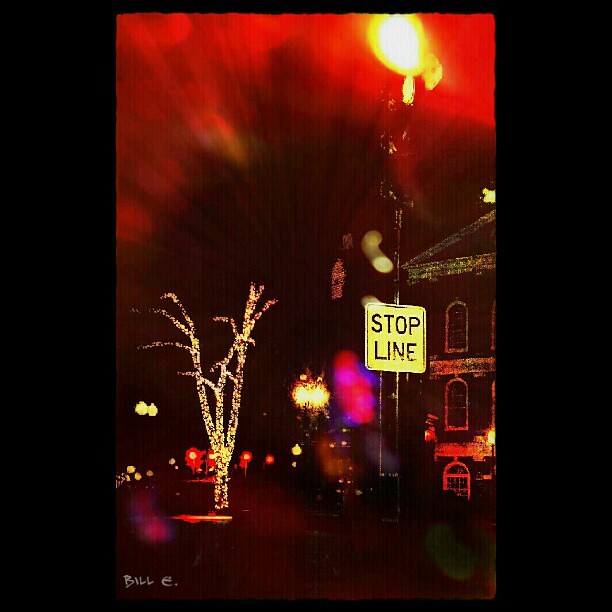This striking image, potentially manipulated or painted over for dramatic effect, captures a colonial-style building on the right with arched windows and vintage brick architecture. A streetlight with a "Stop Line" sign stands prominently next to it. The scene is awash with glowing streetlights and a tree adorned with miniature Christmas lights, adding a festive touch to the composition. The night sky, vividly red, creates an almost surreal backdrop with rays or lines appearing to shoot upwards, possibly due to the camera's prolonged exposure capturing every detail of light. These anomalies give the image a unique, overexposed look, highlighted further by the photographer's name, Bill E., inscribed at the bottom left. The overall effect is a visually spectacular, almost otherworldly night scene.